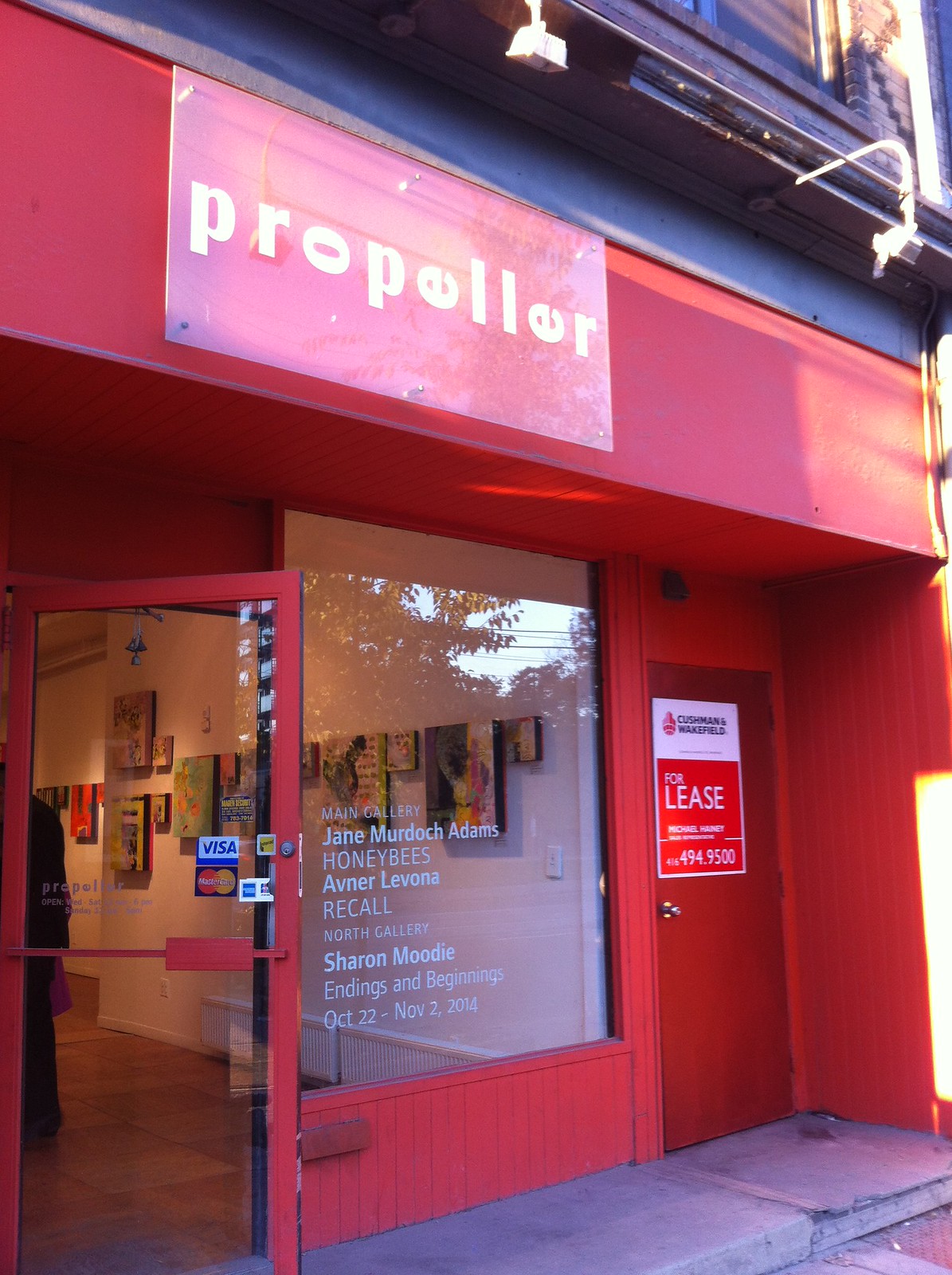The storefront of the gallery named "Propeller" is distinctively painted red and features a prominent sign at the top. The sign reads "Propeller" in white font, with the E's and last O rotated 90 degrees upward, giving it a unique and artistic appearance. The storefront includes a large glass window and a glass door, both of which have various writings and stickers, including Visa and MasterCard logos, indicating the acceptance of credit cards.

On the window, a list of names and details of an exhibition catch the eye: "Main Gallery, Jane Murdoch Adams, Honeybees, Avenir, Livona, Recall, North Gallery, Sharon Moody, Endings and Beginnings, October 22nd to November 2nd, 2014." Through the glass, several paintings can be seen hanging on the white walls of the interior, suggesting the place is an art gallery.

To the right of the main window, there is a closed red-painted metal door with a "For Lease" sign on it, hinting that the space might be part of a larger strip of businesses. The ground outside the gallery is a cement sidewalk, while inside, the floor consists of brown tiling. The storefront is visually accessible, with a few glimpses of people inside, contributing to the gallery's lively and welcoming atmosphere.